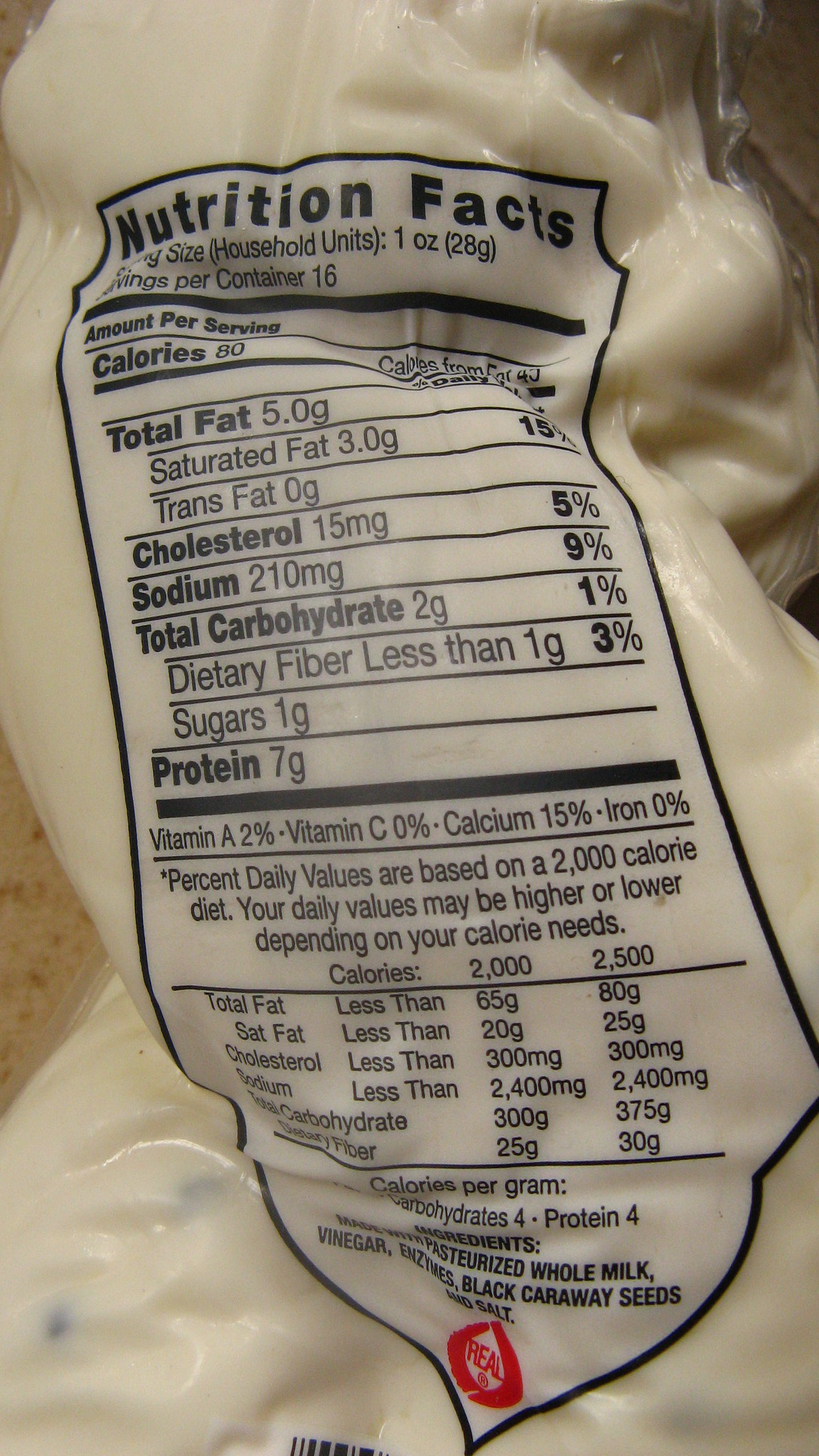This photograph, taken in portrait orientation, depicts the back side of a vacuum-sealed plastic container filled with cheese curds containing black caraway seeds. The plastic packaging is not see-through, and it features a detailed nutritional label printed in black font on a stark white background. The label confirms the ingredients as whole pasteurized milk, vinegar, enzymes, black caraway seeds, and salt, indicating it is indeed cheese with caraway seeds. Prominent on the label is a red circular "Real" symbol, certifying the product as genuine dairy. The nutrition facts section reveals that each of the 16 servings contains 80 calories, with a breakdown of total fats, saturated fats, trans fats, cholesterol, sodium, carbohydrates, dietary fibers, sugars, protein, and various vitamins and minerals. The detailed black-and-white label provides essential dietary information, emphasizing that daily values are based on a 2,000 calorie diet. Sealed in its container, the cheese exhibits a white, slightly gooey texture with visible black caraway seeds.